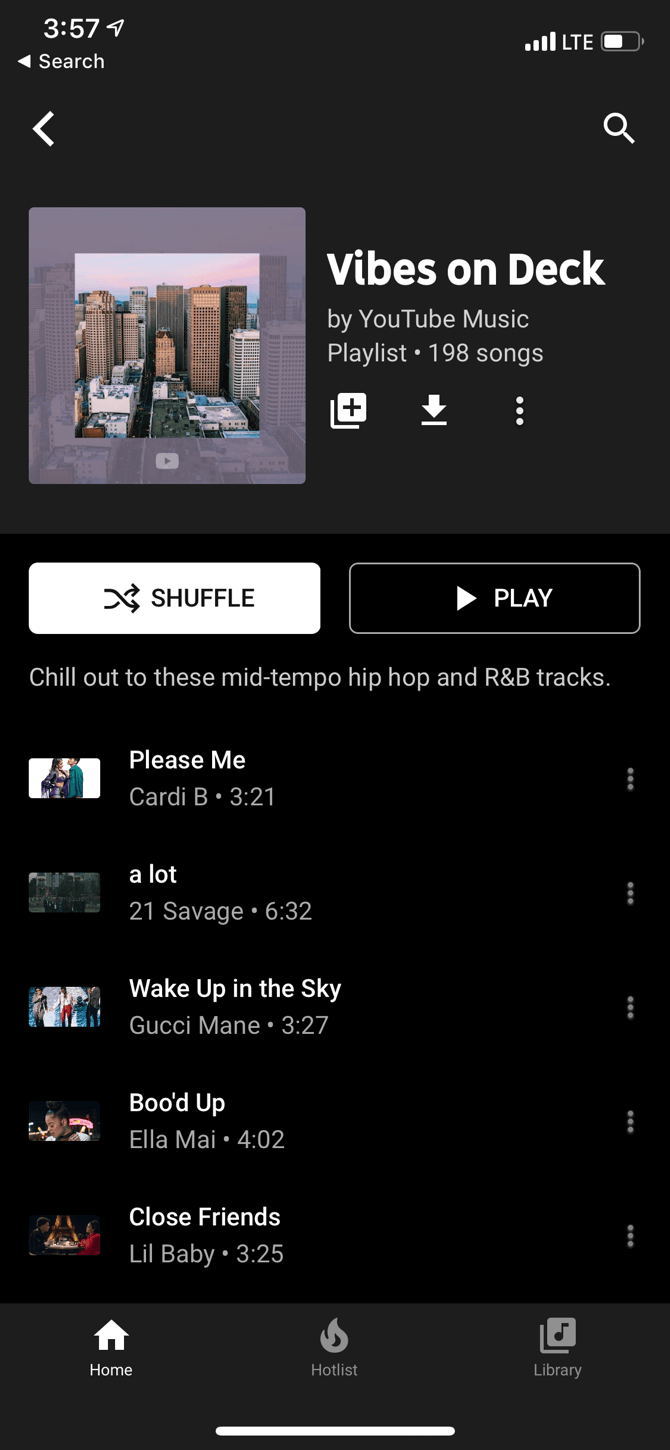The image is a screenshot of a YouTube Music playlist titled "Vibes on Deck." The playlist consists of 198 songs and is tailored to those who enjoy mid-tempo hip-hop and R&B tracks. At the top of the playlist, the title "Vibes on Deck" is prominently displayed with the label "by YouTube Music" beneath it.

To the left of the playlist information, there is an image of a cityscape, which adds a visual element to the theme. The middle section of the screen features two buttons: "Shuffle" and "Play," allowing users to either listen to the playlist in a random order or sequentially from the beginning.

Some of the featured tracks in the playlist include:

- “Please Me” by Cardi B
- “A Lot” by 21 Savage
- “Wake Up in the Sky” by Gucci Mane
- “Boo’d Up” by Ella Mai
- “Close Friends” by Lil Baby

Each song is accompanied by its respective cover art, enhancing the visual appeal of the playlist.